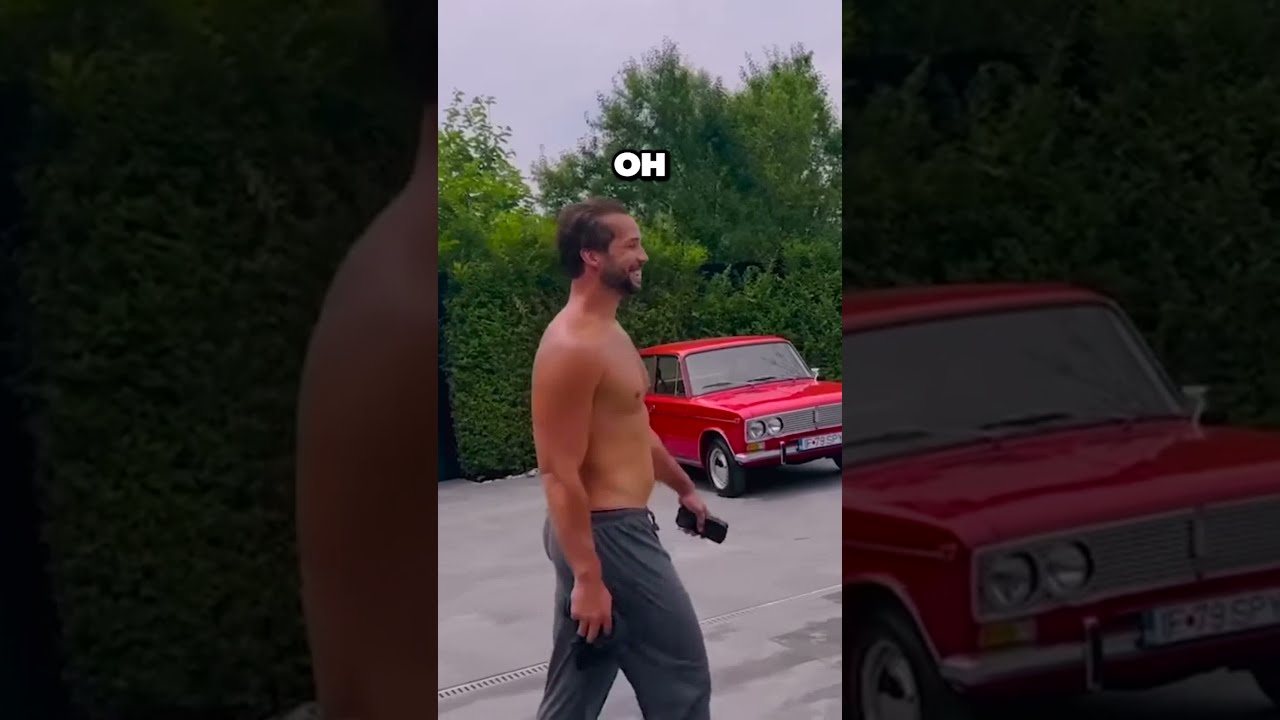The image captures a shirtless young man with a medium tan, a beard and mustache, and short brown hair, walking in a parking lot or driveway area. He is wearing dark gray sweatpants and is viewed from a side profile, smiling and holding a cell phone in his left hand. The background features a bright red vintage-looking car with a European or Russian license plate, which appears to have been parked there for some time. The parking lot is paved with asphalt and equipped with a rain gutter. Behind the car, green hedges and trees are visible, although one tree seems in need of trimming. Above the man's head, the letter "O" is displayed in white text, and the overall atmosphere hints at a warm day despite cloudy skies.